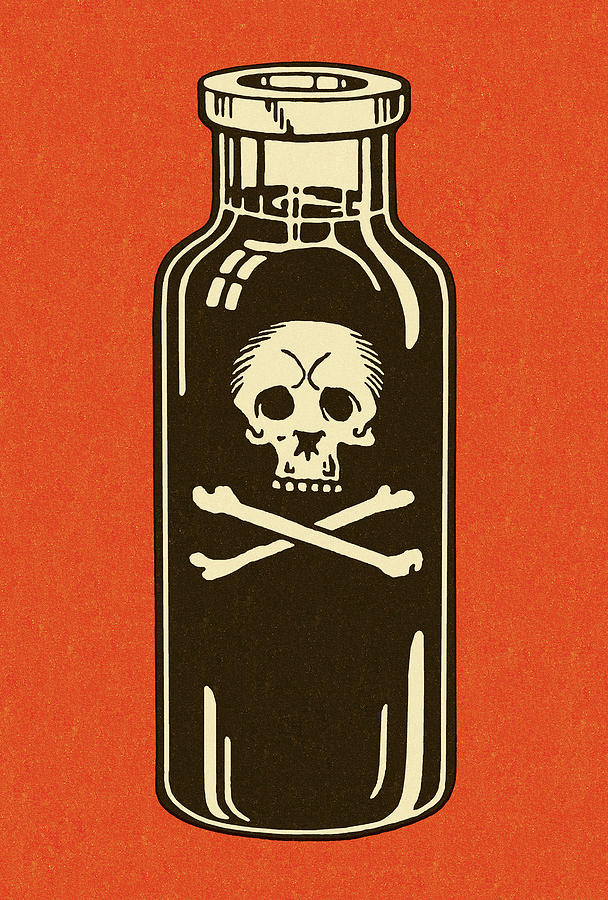This color illustration features a crystalline glass bottle filled with a black liquid, prominently placed in the center against a vibrant orange background. The bottle, which occupies approximately 75% of the frame, is adorned with a stark skull and crossbones emblem indicating its poisonous content. The bottle is detailed with white lines to suggest reflections or a light source, emphasizing its three-dimensional form. At the top, the bottle has a cap with a hole cut into it, adding to the eerie atmosphere of the image. The illustration, devoid of any text, people, animals, buildings, or additional objects, emphasizes the ominous nature of the bottle and its deadly contents.